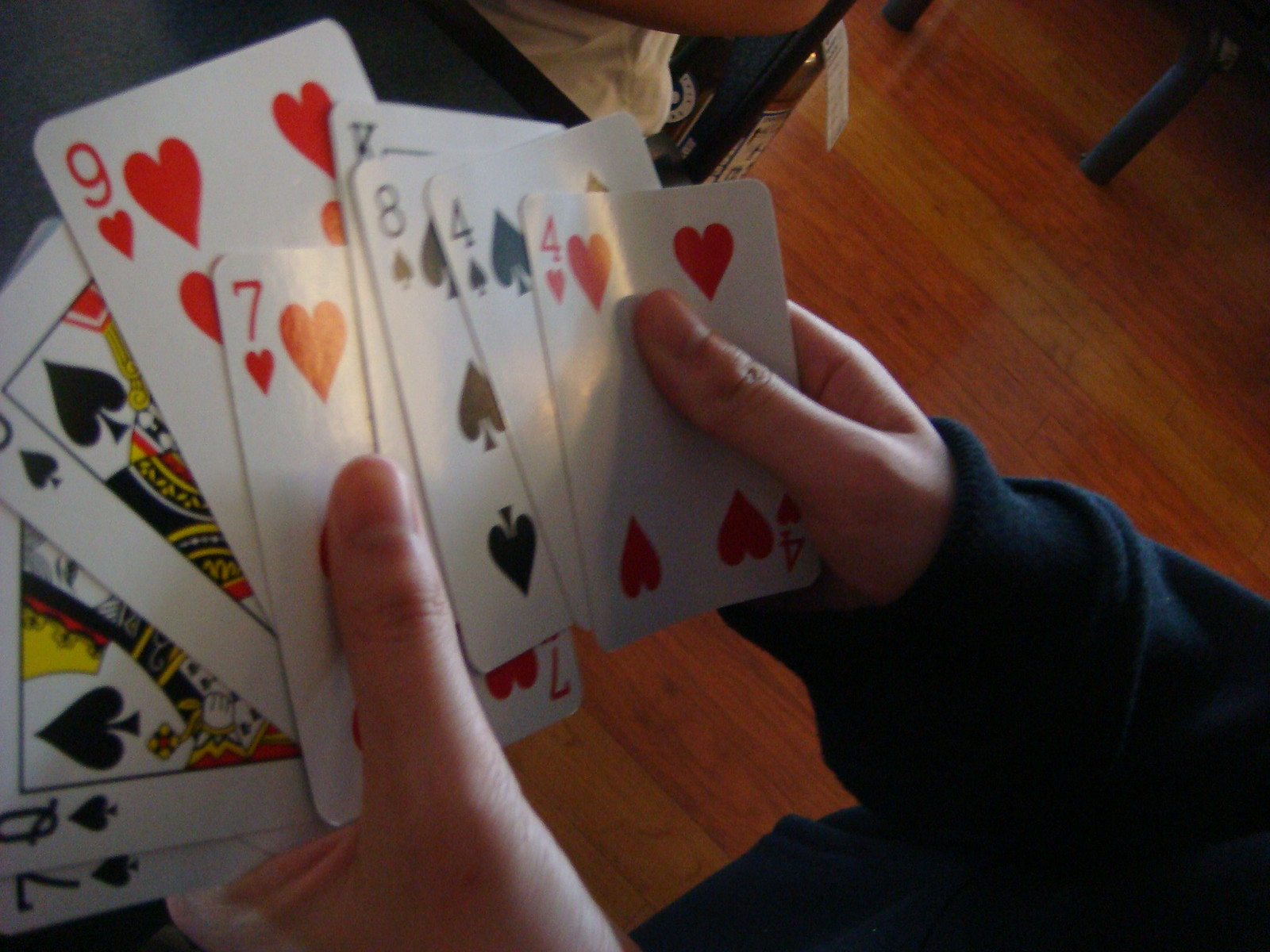In this detailed image, a white male is seated at a table with a black surface, inside a room that features a finished brown floor with yellowish undertones. He is wearing a black hoodie and is holding several playing cards that appear to have been dealt to him. To his right, someone else is also seated, partially visible.

The cards in his hand are held in a fanned arrangement, moving from right to left. The first card is the black 7 of spades, displaying an upside-down heart and stem, characteristic of the spades suit. Next, the Queen (Q) of spades is partially visible, adorned with a detailed figure in the center, and highlighted with colors such as yellow and red. The following card, although unclear if it is another Queen (Q) or a different rank, is also of the spades suit, featuring both small and large spade icons.

Additionally, he holds the red 9 of hearts, showing the number 9 on the top left corner and two heart symbols. Another card, the 7 of hearts, is also visible, colored red, with one heart beneath the number 7 and another adjacent. Among his fan of cards, there is also a King (K), an 8 of spades, a 4 of spades, and a 4 of hearts, each distinctly marked with their respective suits and numbers.